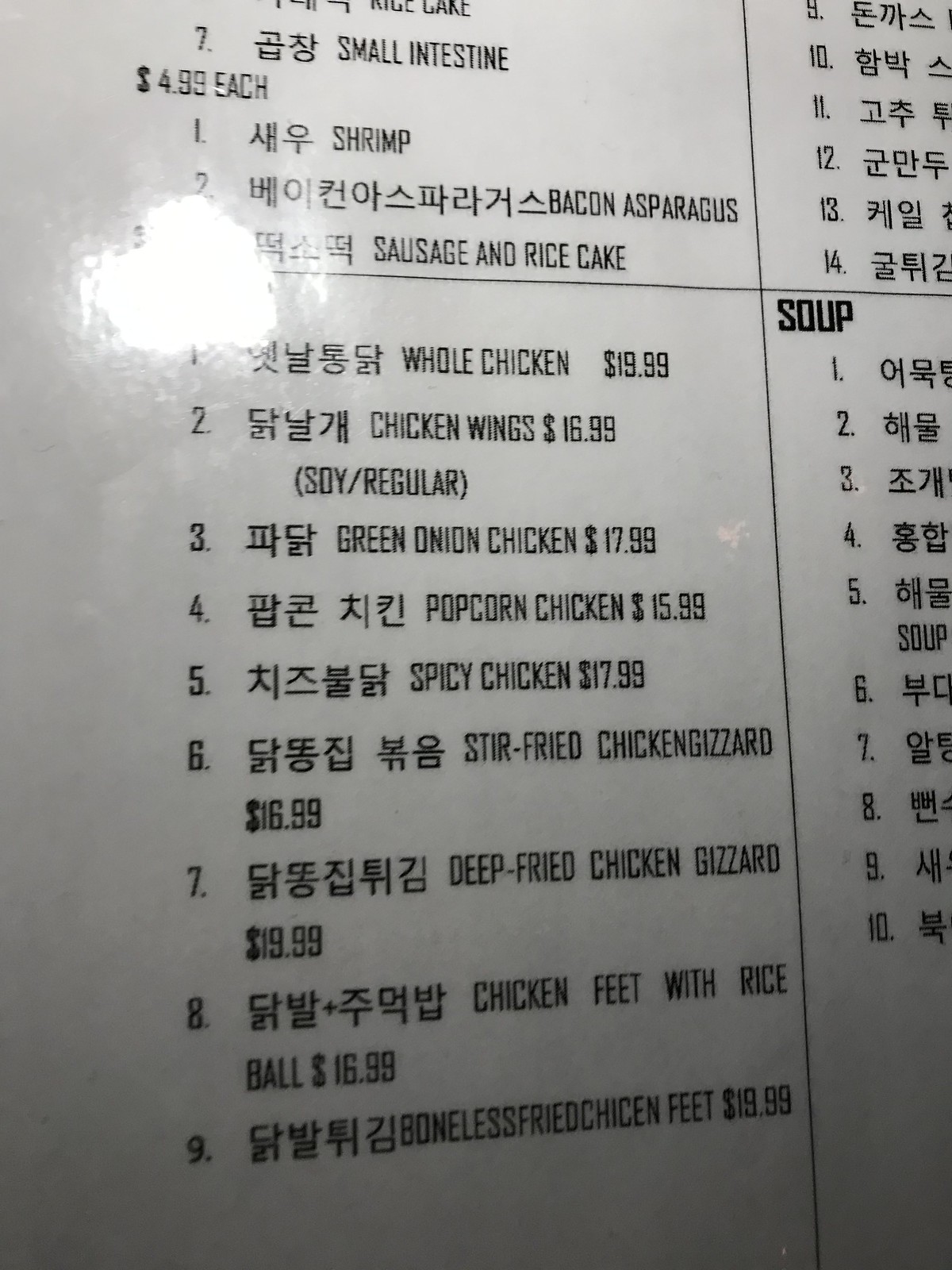This image depicts a laminated white menu with a bright reflection that obscures some of the items. The menu appears partially visible, with significant portions cut off. At the top of the visible section, the menu begins with the number seven, followed by a Chinese symbol and the English text "small intestine." Below that, the menu is divided into four sections by horizontal lines. The numbering restarts, listing items from one to nine, each with a corresponding Chinese symbol and English translation.

The listed items in English are as follows:
1. Whole Chicken - $9.99/$19.99
2. Chicken Wings - $16.99 (described as "soy irregular")
3. Green Onion Chicken - $17.99
4. Popcorn Chicken - $15.99
5. Spicy Chicken - $17.99
6. Stir-Fried Chicken Gizzard - $16.99
7. Deep Fried Chicken Gizzard - $19.99
8. Chicken Feet with Rice Ball - $16.99
9. Boneless Fried Chicken Feet - $19.99

In the top right corner, items numbered 9 through 14 are partially visible, showing only the Chinese symbols. Below this, there is a section labeled "Soup," which lists items numbered 1 through 10, though only some Chinese symbols are visible due to the cutoff.